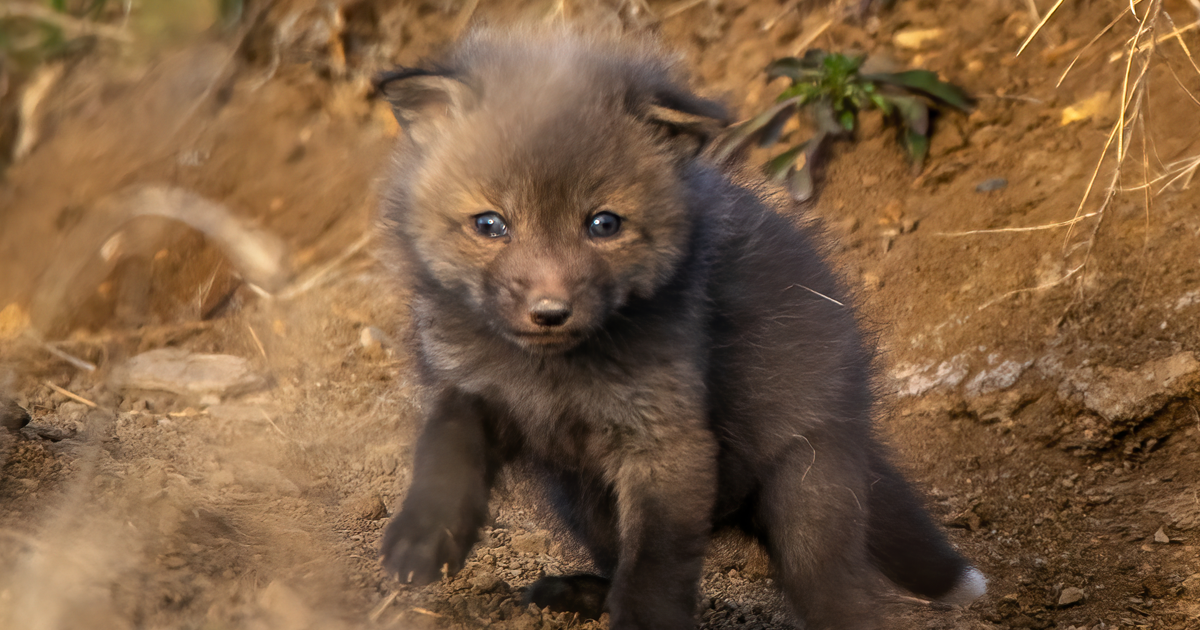This color photograph captures an incredibly cute baby animal nestled in earthy red dirt. The little creature's brown and grayish-black fur appears fluffy and well-groomed, framing its adorable blue eyes and tiny pointy nose. Although its exact species is indeterminate—possibilities include a wolf pup, coyote pup, or even a baby bear—the animal certainly exudes a wild charm with its sharp claws and prominent pointy ears. Its small, folded ears and white-tipped tail add to its irresistible cuteness. The setting features uneven terrain with dirt, scattered stones, and patches of green weeds growing in various directions. In the background, some brown sticks or grasses are visible, blending into the natural, rugged landscape.